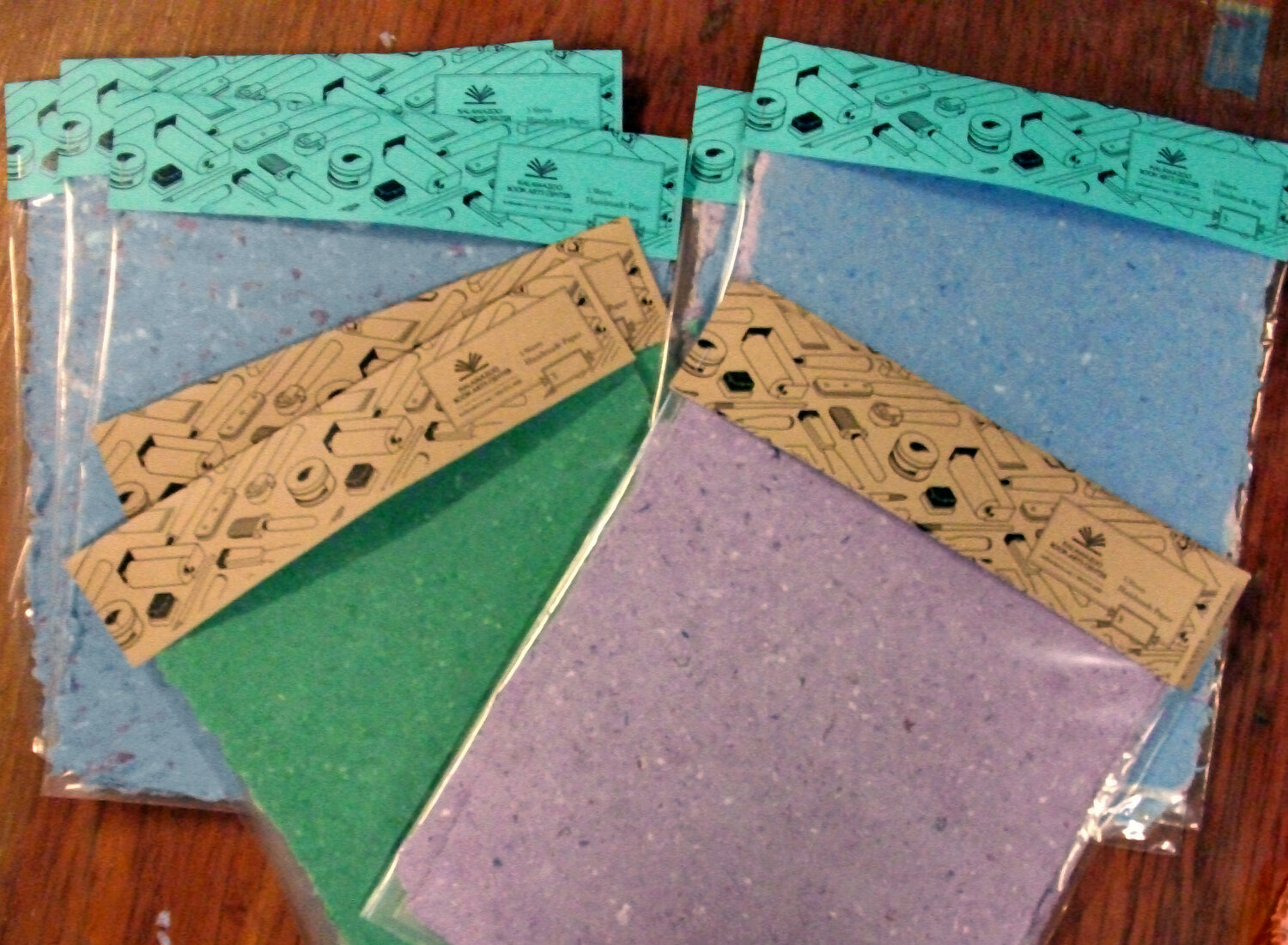The image depicts a somewhat blurry, amateurishly taken photo featuring stacks of clear polybags, each containing fabric swatches or flat materials of various colors. The polybags are arranged on a dark hardwood floor or a brown table, with two distinct stacks, each containing three or more swatches. The swatches inside the polybags are square-shaped and come in colors of baby blue, dark green, and light lavender or mauve. These packaged swatches have paper labels at the top, with black ink writing and illustrations that seem to depict construction and painting tools. The labels for the green and mauve swatches are tan-colored, while the labels for the blue swatches are cyan.